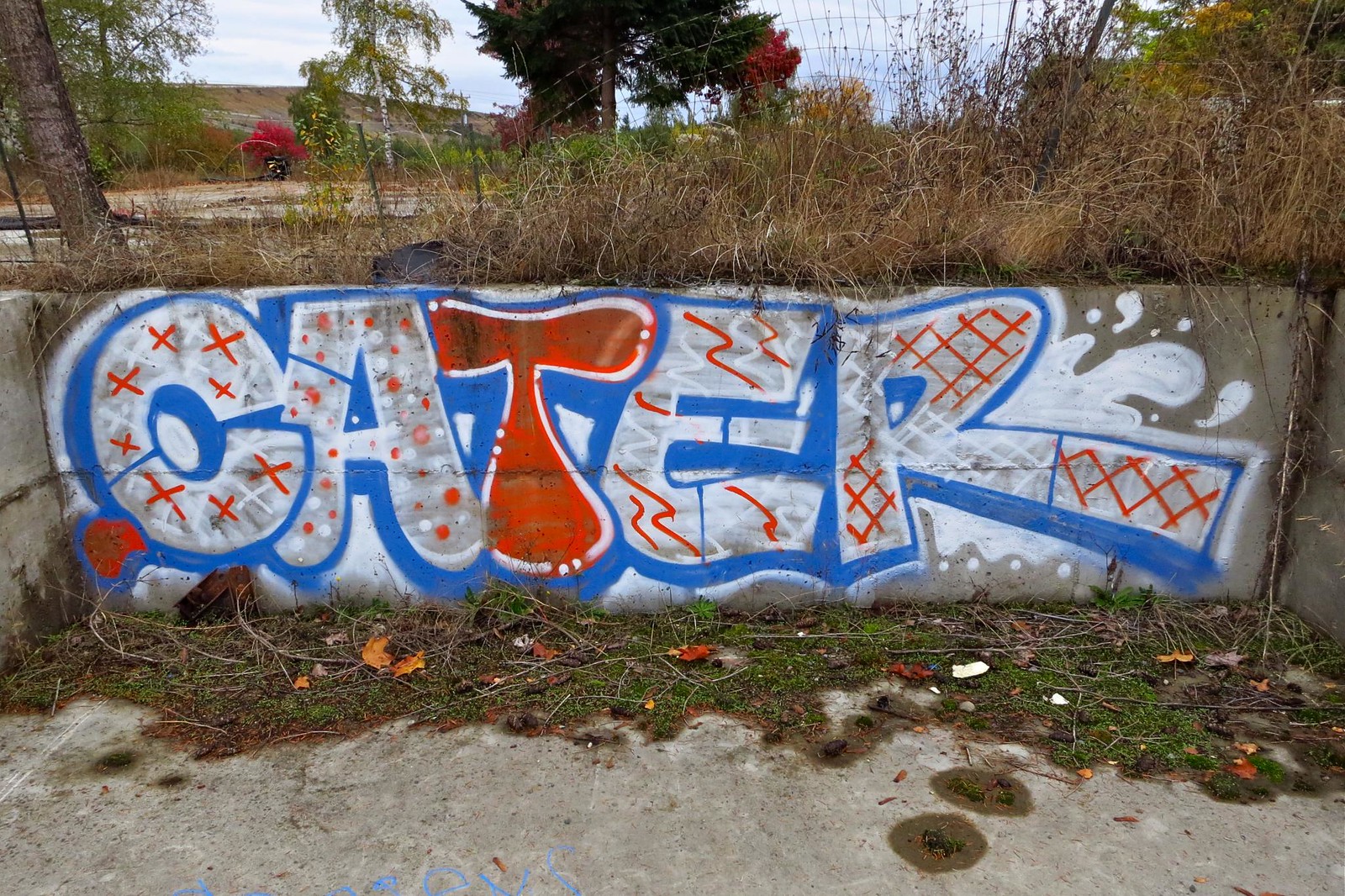The photograph captures a vibrant piece of graffiti situated in what appears to be a concrete drainage ditch or retaining wall. The sky visible at the top of the image is light blue with multiple clouds, suggesting a bright daytime setting. In the foreground, there is a gray asphalt surface within a concrete cubby area, dotted with damp spots, grass, fallen branches, and roots. This area is sunken in, about two feet deep, reinforcing the impression of a drainage ditch or similar structure. 

The graffiti itself is a striking display of the word "CATER" in large white letters, each accented by a blue outline. Notably, the letter "T" stands out with an orange fill and a white border. Each letter is intricately detailed: the "C" features red and white X marks, the "A" is adorned with red and white dots, the "E" has small red and white wiggles, and the "R" displays a red and white cross-hatch pattern. The background includes a deserted field with grass, shrubs, and scattered trees. A road and a vehicle are faintly visible in the upper background, adding depth to the open, outdoor setting. The overall scene is detailed with hints of nature reclaiming the area, juxtaposed against the vivid and artistic graffiti.